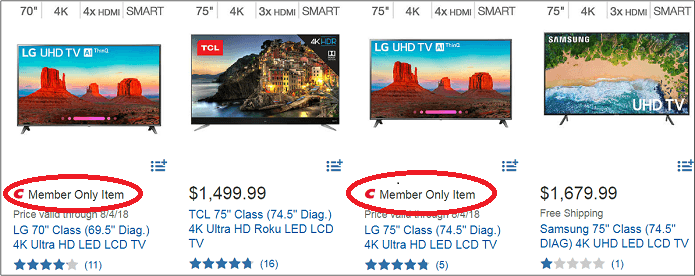A rectangular advertisement leaflet is outlined in black, featuring a gray vertical line dividing the content into four sections. Each section contains information about different smart TVs, structured as follows:

- The first section lists:
  - "70 inch 4K 4x HDMI Smart" and displays an image of an LG UHD TV.
  - A paragraph below the TV image states: "Member-only item, price valid through 04/18," followed by "LG 70 inch Class Ultra 4K," with a four-star rating.

- The second section lists:
  - "75 inch 4K 3x HDMI Smart" and displays an image of a TCL TV.
  - A paragraph below this TV image shows a price: "$1,499.99," accompanied by a five-star rating.

- The third section lists:
  - "75 inch 4K 4x HDMI Smart" and displays an image of another LG UHD TV.
  - A paragraph beneath this TV image mentions: "Member-only item," with a five-star rating.

- The fourth section lists:
  - "75 inch 4K 3x HDMI Smart" and features an image of a Samsung UHD TV.
  - A paragraph below this TV image shows a price: "$1,679.99," specifies "Free shipping," and includes a one-star rating.

This detailed layout succinctly highlights the key features, brands, member specifics, ratings, and pricing for each TV model.